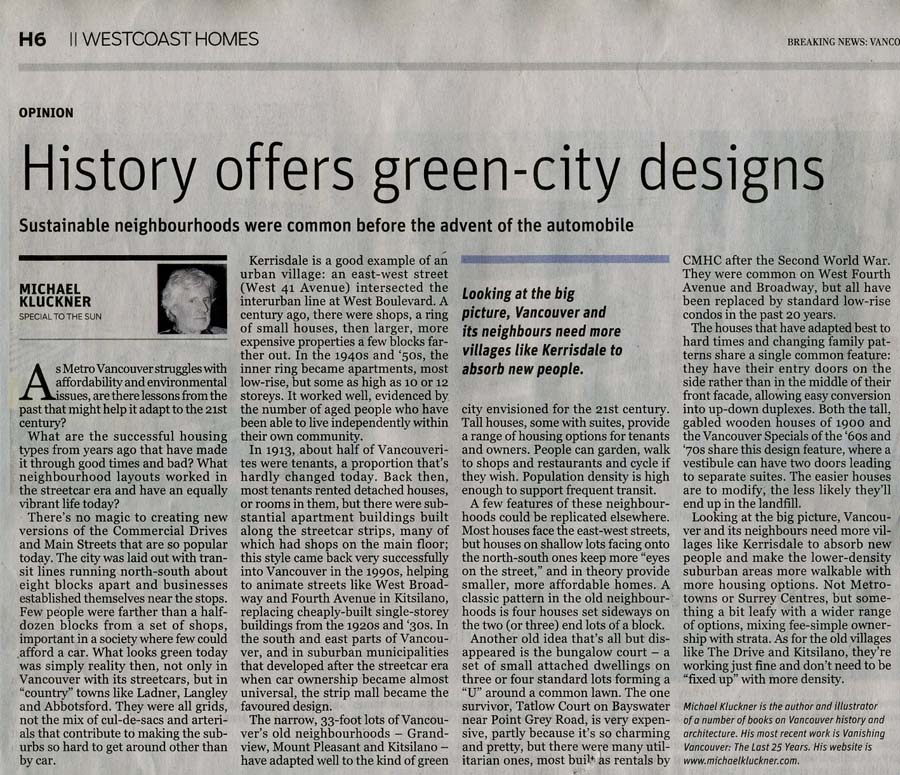The photograph depicts a page from a newspaper, likely a publication based in Vancouver, given the context of the article and a truncated "Vanco" visible in the breaking news section at the top right. The top left of the page displays "H6" and "Page, West Coast Homes." The main feature is an opinion piece by Michael Kluepner, titled "History Offers Green City Designs, Sustainable Neighborhood." The article discusses historical urban design principles, which were prevalent before the advent of the automobile, advocating for more sustainable city planning.

The piece spans four columns from left to right. Within the text, there's a significant excerpt highlighting the article's focus: "Looking at the big picture of Vancouver and its neighbors in more villages like Kersdale, absorbing people," suggesting that the suburb of Kersdale might be central to the author's argument about sustainable neighborhoods.

The newspaper itself has a typical gray and white background with black ink. Notably, a blue bar is present above the mentioned excerpt, indicating some use of color on the page. The overall layout and design reflect a standard newspaper format with minimal visual elements beyond the essential text and occasional highlights for emphasis.